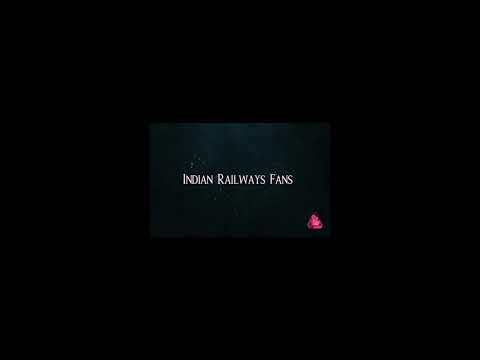The image is a graphic advertisement presented in a landscape-oriented rectangular frame. Dominated by a black background, it subtly reveals a light grayish band just above the text. In the center of the composition rests a smaller, centered rectangle which hosts the main content. The text "INDIAN RAILWAYS FANS" is prominently displayed in crisp, all-uppercase white lettering towards the bottom right of this central rectangle. Just two-thirds of the way to the right within the frame, there's a distinctive bright pink logo resembling a squiggle or a flame. The overall design incorporates elements of black, white, and bright pink, though its understated color scheme might not immediately catch the eye.